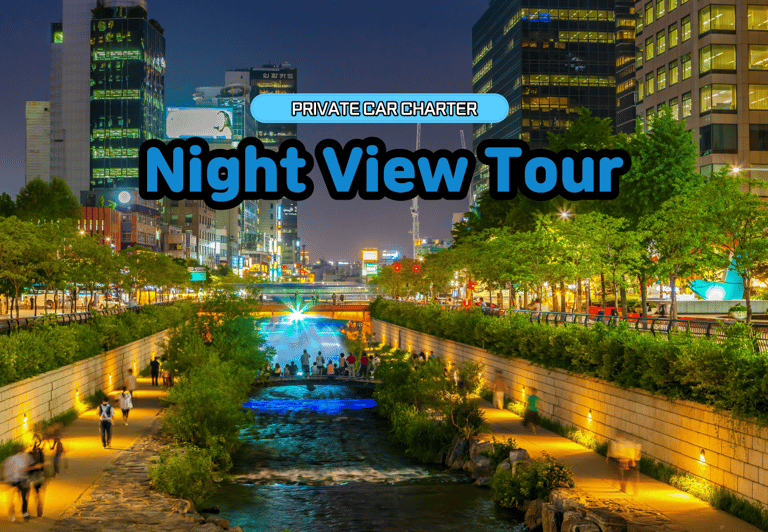The image depicts a bustling cityscape at night with a prominent sunken walkway alongside a river that runs through the scene. The walkway, which features short trees and bushes, is flanked by high walls on either side, dividing it from the upper-level promenade and regular streets. Pedestrians stroll along the illuminated path, which is beautifully adorned with orange and yellow lighting. The river itself includes a large, captivating blue fountain at its center. Various bridges connect different levels of the promenade, including a footbridge crossing the river. In the background, tall buildings, likely business or residential skyscrapers, frame the dusky blue to purple night sky. Adding a touch of modernity, a train trestle with motion-blurred trains and a platform with waiting passengers can be seen. Superimposed over this vibrant urban scene is a color block displaying the text "Private Car Charter" in white font and "Night View Tour" in blue font, bordered by thick black lines, suggesting perhaps that this is an illustration or rendering of a proposed city area meant for promotional purposes.